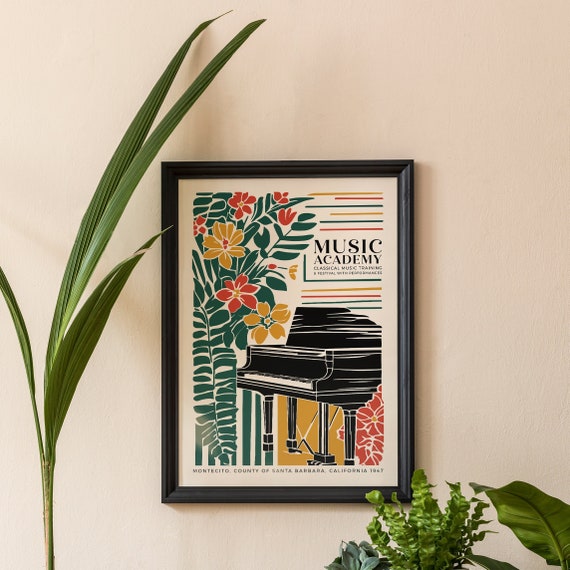The image depicts a beige or tan-colored wall adorned with a vintage, black-framed poster. The poster features an illustration of a black piano, encircled by an array of vibrant flowers and foliage. To the left of the piano, lush green leaves stretch above it, with golden-yellow and red flowers intertwined among the branches. On the right, more flowers emerge in similar hues. The poster prominently displays the phrases "Music Academy" and "Classical Music Training and Festival with Performance" in bold black letters across the top. At the bottom, additional text reads "Montecito, County of Santa Barbara, California, 1947," suggesting a historical or commemorative significance. Real, long-leafed plants also surround the wall, enhancing the room's decor with a natural touch.